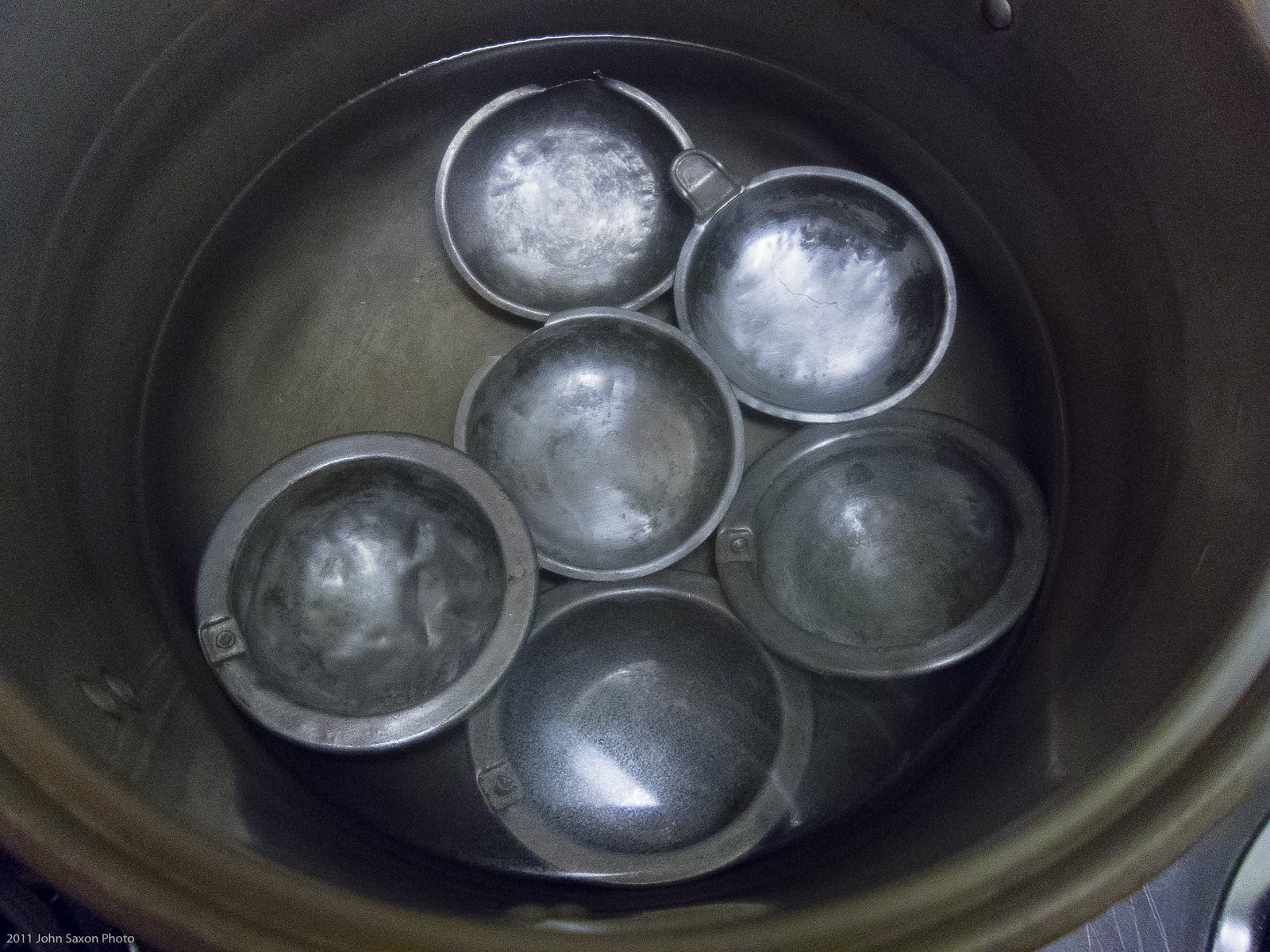The photograph captures an aerial view of a deep, olive green bucket containing a round, large metal tray at its base. Arranged meticulously side-by-side on this tray are six relatively flat, shallow metal bowls, reminiscent of dog food dishes. The bowls, possibly made of silver or another gray metal, exude an aged yet well-preserved quality, showing minimal signs of wear. Among the six, one bowl features a burnt spot, while one possesses a handle. Noteworthy, three of the bowls have visible screws indicating where handles once were. The uniform shape and metallic material of each bowl generate a vintage and utilitarian aesthetic.